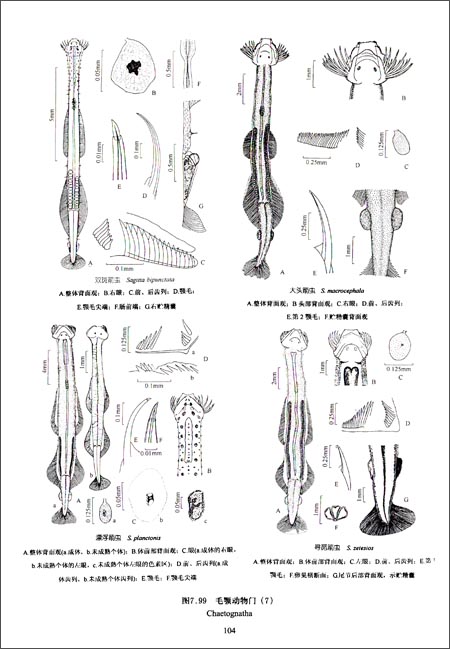The image is a detailed black-and-white scientific illustration, reminiscent of what one might find in a biology textbook or an encyclopedia. It appears to be an in-depth study of different narrow, eel-like organisms, potentially belonging to the Chaetognatha phylum. The page is sectioned into four distinct quadrants, each dedicated to a different species or variant. In every quadrant, the left side showcases the full body of the organism, while the right side includes detailed breakdowns and zoom-ins of various anatomical features—such as the head, lateral fins, tail, and internal structures.

Each detailed diagram is meticulously labeled with text, believed to be in Japanese, including measurements of each body part. The layout also includes cutaways to highlight specific bones or skeletal segments of these fish-like creatures, some of which may appear prehistoric. The entire composition is presented in a portrait orientation on page 104 of the source material.